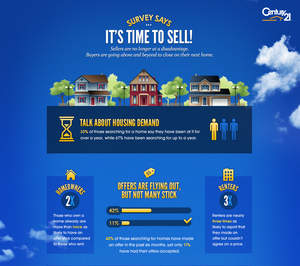This advertisement for Century 21 captures attention with its vibrant royal blue background, interspersed with a few fluffy clouds—some situated in the upper right corner, near the Century 21 logo, and others in the lower left. Dominating the top middle of the ad, the bold text reads, "Survey says: It's time to sell!" with an exuberant exclamation point. Below this proclamation, a row of three charming houses is depicted, each bordered by trees and street lamps, creating a picturesque neighborhood scene.

To the right, an hourglass visually emphasizes the urgency with the phrase, "Time is running out," followed by "Talk about housing demand." Below this, three human silhouettes are shown, with one illuminated in yellow to signify its distinction from the two blue figures beside it.

Further down, the caption "Offers are flying out but not many stick" highlights the competitive nature of the housing market. A graphic of a ticket displays a 42% and 11% figure with a checkmark, likely indicating offer acceptance rates. At the very bottom, two circular symbols appear within rectangles on either side— the left one displaying "2x" and the right one "3x"— possibly denoting a multiplier effect related to the market conditions or selling power.